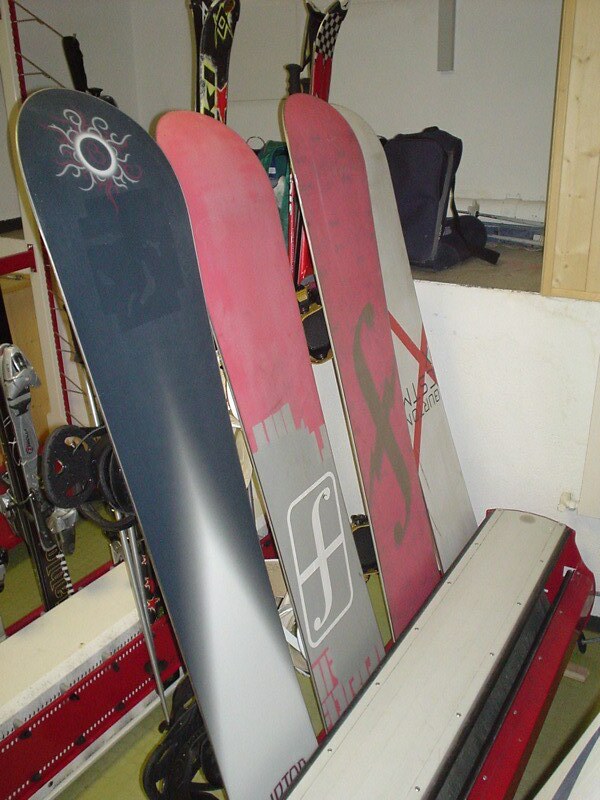The image displays a collection of snowboards and skis, likely taken inside a winter resort, ski shop, or repair shop. The focus is on the bottom parts of four snowboards, each featuring distinct designs and colors. The first snowboard is predominantly black with a white sun emblem. The second is red at the top and gray in the middle, sporting a white 'F' logo. The third board is entirely red, also marked with a similar 'F' logo, but in brown, suggesting it may be from the same brand as the second. The fourth snowboard is all gray with red lettering and a red 'X'. In the background, a row of skis is visible, hanging from the wall. These skis include one with a black, white, and red checkered design and various others with less distinguishable patterns. The scene suggests an organized display, possibly for rental or sale, supported by some wooden beams and a red and white stand that holds the equipment securely. Overall, the image captures a neatly arranged indoor setup of snowboards and skis against a wooden backdrop.